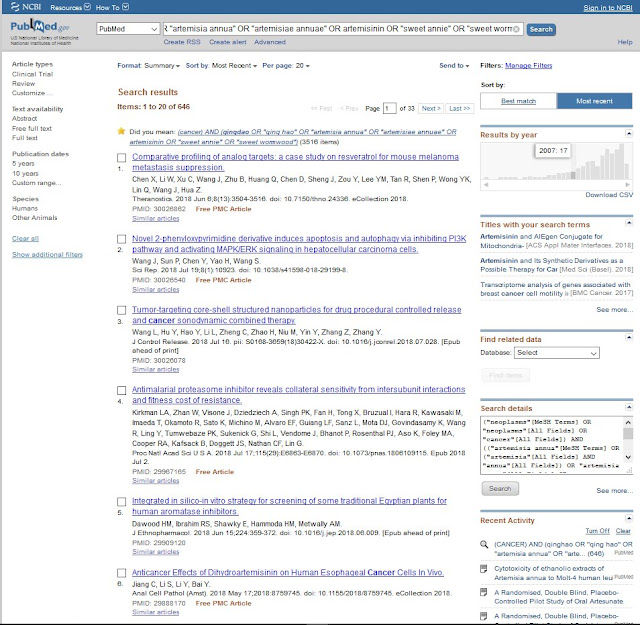The image depicts a webpage from PubMed.gov, a platform operated by the National Center for Biotechnology Information (NCBI). The page is dominated by a search box located at the top, inviting users to enter key medical terms for retrieving relevant articles. Designed much like a specialized search engine, PubMed offers several filter options to refine search results, including article types (such as clinical trials and reviews), text availability (like abstracts, free full-text articles, and full-text articles), and publication dates (with options like the past five years, ten years, and custom date ranges).

The search results on this example page are numbered from 1 to 20, out of a total of 646 results. Additionally, there is a bar graph depicting the distribution of search results over time, highlighting an entry for the year 2007 with 17 results. The graph shows a general increase in the number of results as the years progress. Each search result is accompanied by titles and other relevant data, aiding users in quickly identifying pertinent information.

On the right side of the page, there is a section labeled "Recent Activity" that provides key insights based on recent searches. The overall design of the webpage features a primarily white background, with blue accents at the top and a gray-shaded search section to help differentiate the search functionalities.